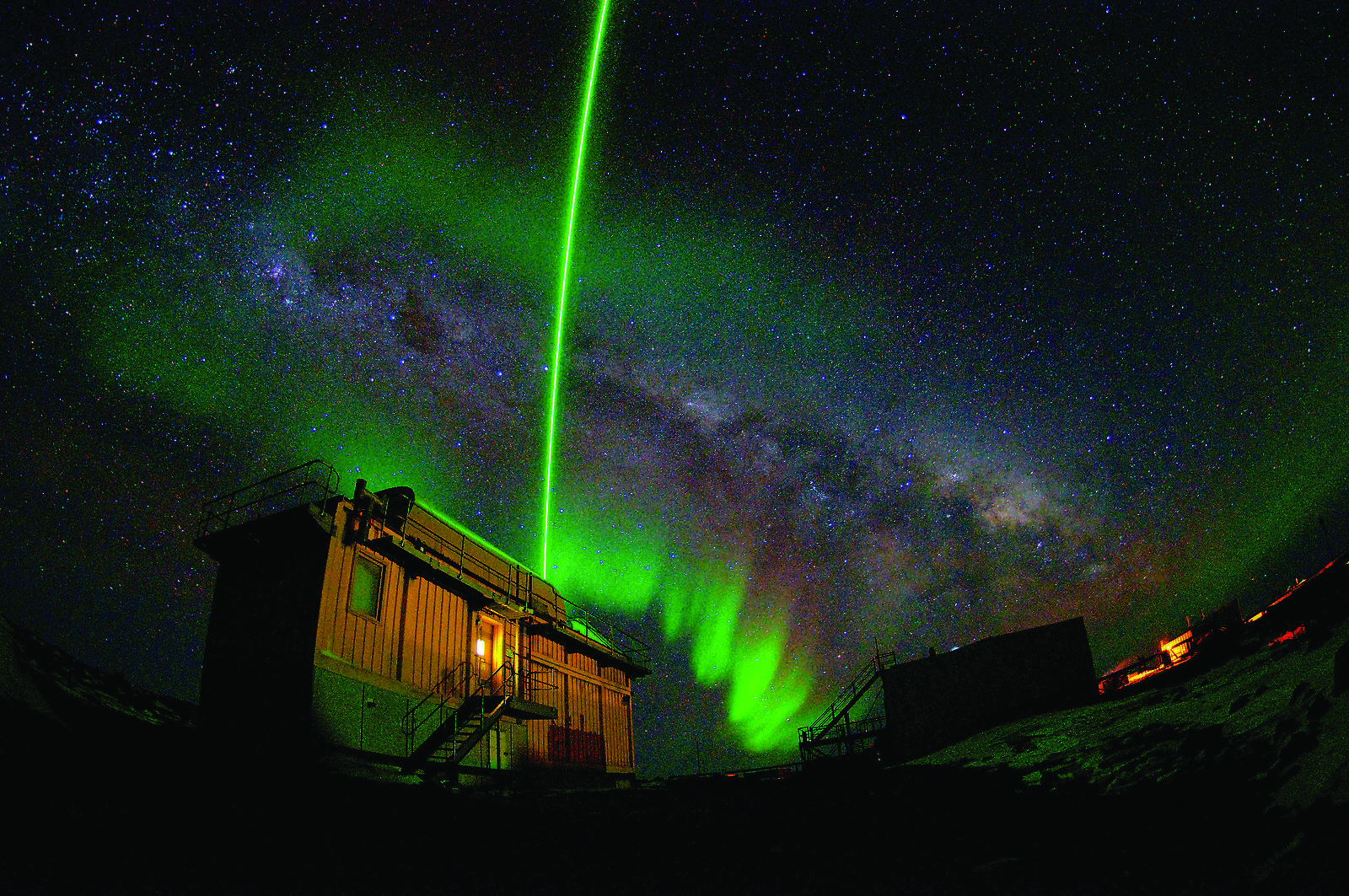The photograph captures the mesmerizing Aurora Borealis, or Northern Lights, against a dark, star-speckled night sky. The celestial display features a vibrant green aurora prominently in the lower left corner, with streaks of lime green light shooting upwards, illuminating part of the scene. A brown building, reminiscent of a vintage train caboose, occupies the lower left corner. This building, bathed in a yellow glow, features a metal staircase leading up to its door and resembles an observation station. To the lower right, there are additional structures likely part of a scientific or observation base. The ground beneath these buildings appears rocky, adding to the remote and rugged feel of the setting. The overall image is both dark and vividly colorful, highlighting the bright green aurora and twinkling blue stars, creating a striking contrast against the night sky. The image is clear and detailed, with no people, words, or numbers visible.